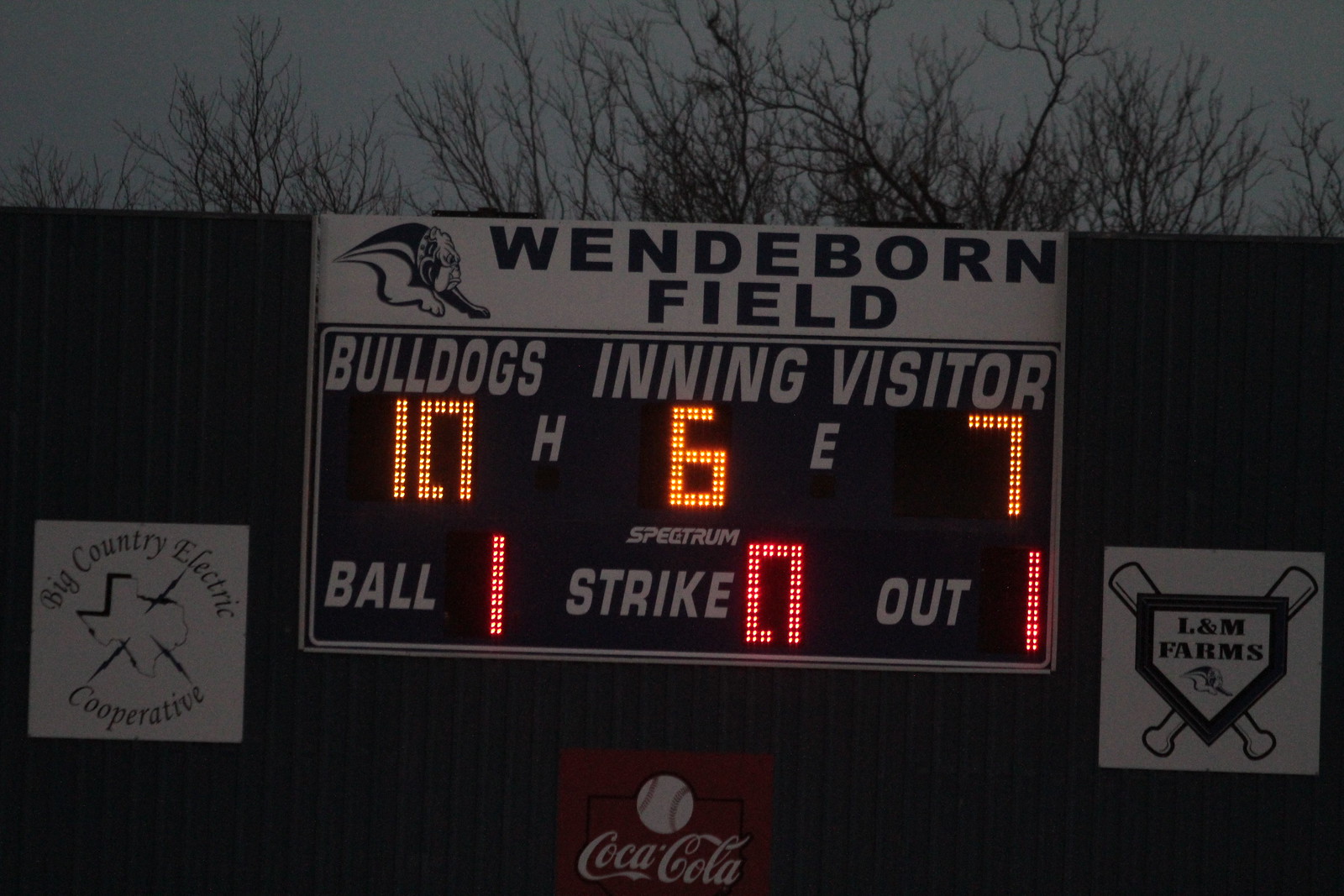This detailed photograph captures a brightly lit scoreboard for a baseball game at Wendy Bourne Field (mentioned alternatively as Wendaborn Field). The scoreboard, mounted on a large black or dark green wall, showcases the scores with illuminated LCD displays in red and yellow colors. The text on the scoreboard reads "WENDY BOURNE FIELD BULLDOGS INNINGS VISITORS BOWL STRIKE OUT." The digits displayed indicate "BULLDOGS 10," "INNING 6," "VISITORS 7," with "BOWL 1," "STRIKE 0," and "OUT 1." Below the scoreboard, three advertisements are visible: one on the left for "Big Country Electric Cooperative" with a design of Texas and lightning bolts, a Coca-Cola ad prominently in the center, and another for "L&M Farms" on the right. The scene appears to be during the evening or nighttime, as indicated by the dark blue sky and the dry, leafless branches of trees protruding behind the wall. The combination of the scoreboard lights and the advertised brands enhances the overall atmosphere of an ongoing baseball game.